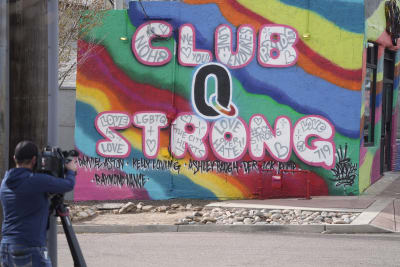The photo captures the vibrant side wall of a building adorned with a large, colorful mural promoting LGBTQ pride. Painted in thick, wavy diagonal bands of rainbow colors—turquoise blue, lime green, red, orange, yellow, light blue, dark blue, pink, and various shades of green—the mural features the prominent white, pink-outlined lettering "Club Q Strong." Each letter houses graffiti-style artwork, with messages of love and pride vividly illustrated, such as the word "Love" inside the letter "S." In the bottom left corner of the image, a man dressed in blue operates a substantial black camera mounted on a tall, sturdy tripod, likely capturing video or photos of the mural. The sidewalk and the continuation of the brightly colored building can also be seen, emphasizing the mural's role in celebrating and supporting the LGBTQ community.